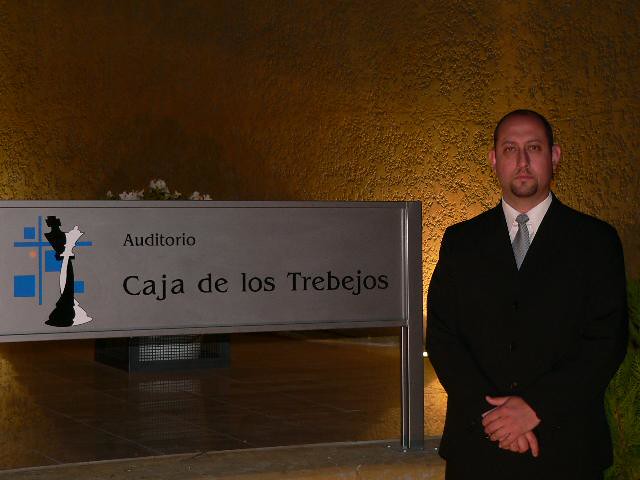In this image, a man is standing on the right-hand side, seen from the waist up. He is dressed in a black suit jacket over a white button-down shirt and a gray tie. The man has very short brown hair and a subtle beard with a faint mustache, giving him a serious expression as he looks directly at the camera with his hands clasped in front of his waist. Next to him, on the left side of the image, there is a metallic grey sign with black letters that reads "Auditorio Caja de los Trevejos" in Spanish. The sign prominently features an intertwined black and white chess piece logo, accompanied by blue lines and squares reminiscent of a chessboard. Behind the sign, part of a statue is obscured, hinting at a historical or perhaps archaeological setting. The backdrop consists of an orange-brown textured stone wall, adding to the dimly lit and possibly cave-like appearance of the environment. The overall scene suggests a solemn and formal atmosphere.